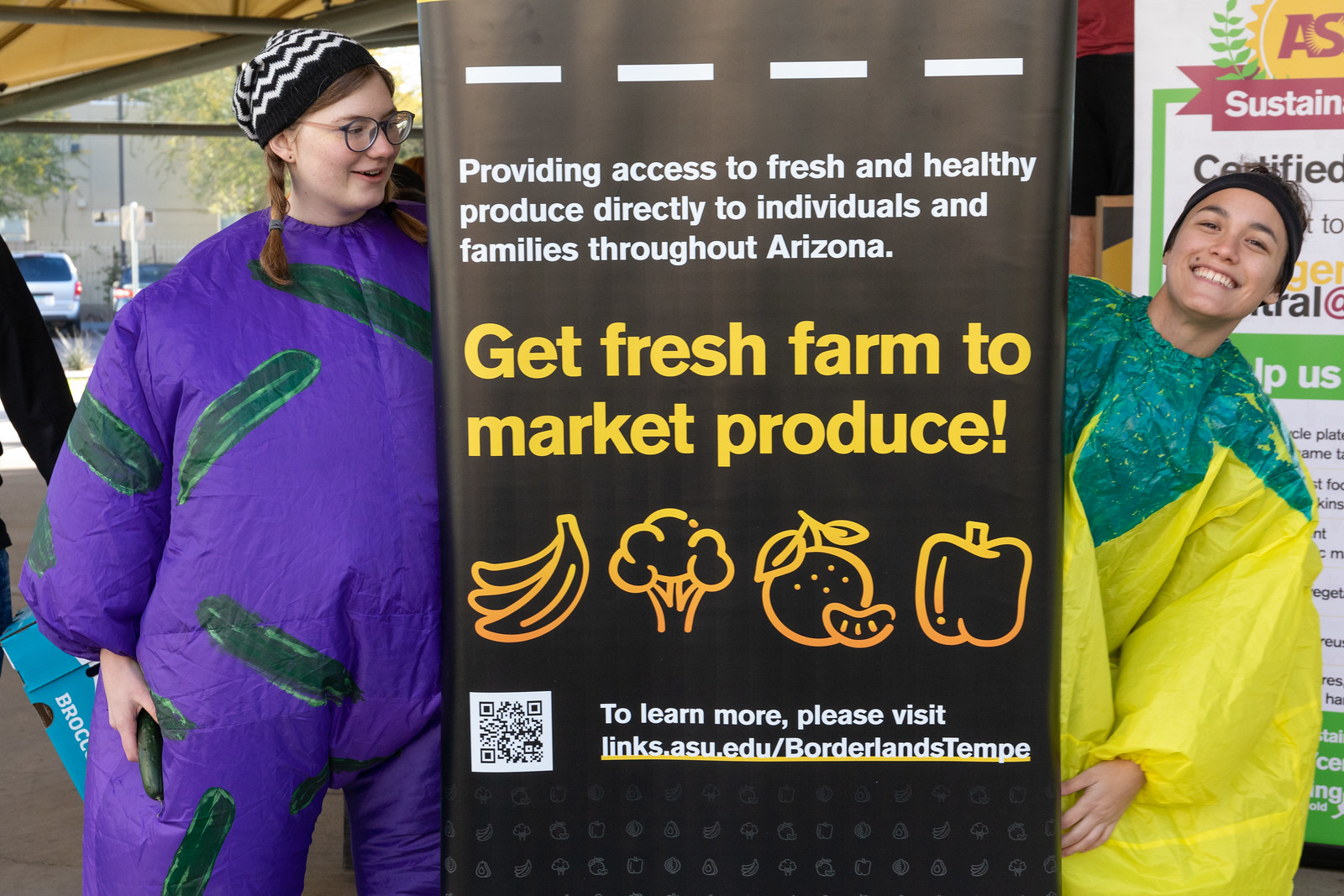In the image, two individuals stand on either side of a brown-backed display that is taller than both of them. The central display features white text reading "Providing access to fresh and healthy produce directly to individuals and families throughout Arizona," followed by yellow text advising to "Get fresh farm-to-market produce." It also showcases iconic pictures of a banana, asparagus, a peach, and an apple. Below this, there is information directing viewers to visit LYNX ASU Education, Borderland Temp for more details.

On the left side of the display, there is a woman dressed in a purple grape-themed costume complete with green fruit designs. She has red hair styled in ponytails, wears glasses, and a ski cap, and holds what appears to be a cucumber. On the right side, there is a person wearing a yellow costume, possibly representing a strawberry, with a green top. This individual, who is smiling, has their hair covered by a headband and is partially obscured by the display.

The background through the glass windows shows a parking lot with cars, suggesting an outdoor setting in a public area, possibly during the middle of the day at a farm fair or similar event. Another banner partially visible behind the person in the yellow costume mentions "sustainable fruit," linking to the overarching theme of fresh produce. The setting features a concrete floor and various colors including purple, green, black, white, tan, and yellow.